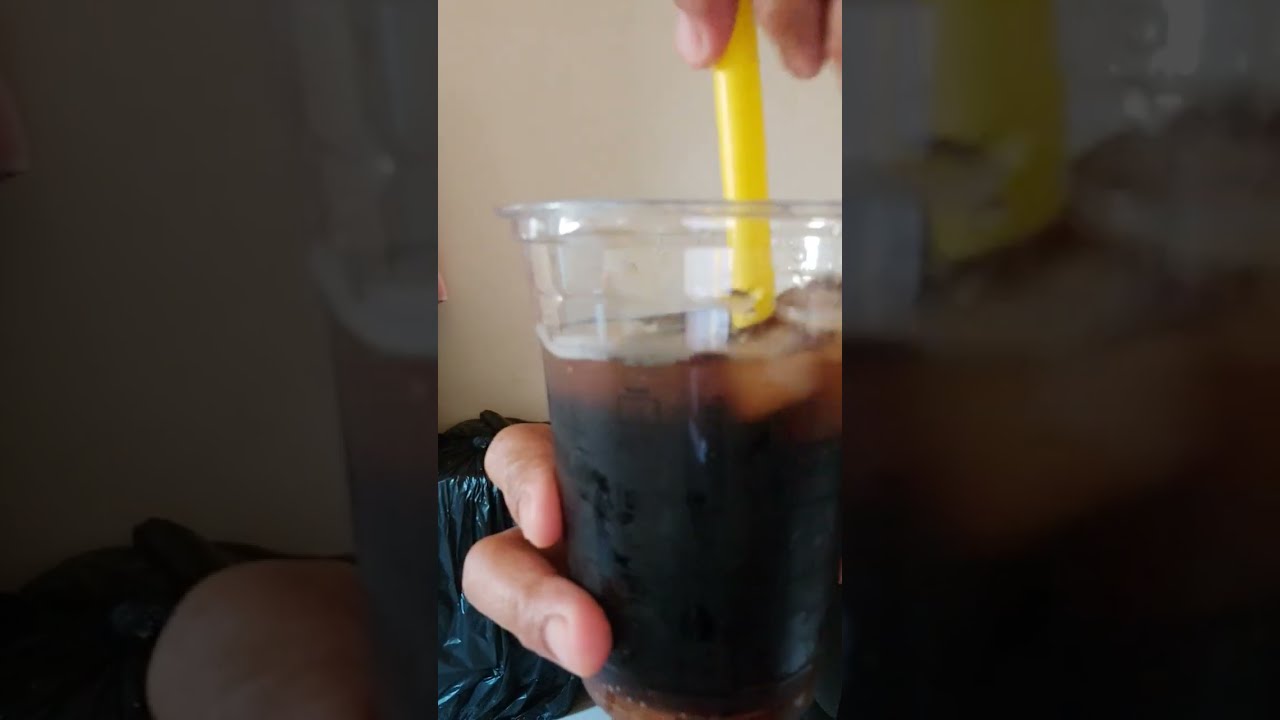The image is divided into thirds, with the central third showcasing an up-close photograph of a nearly full clear plastic glass of dark cola, filled with ice cubes and featuring a yellow straw. The fingers of a white person, with very short trimmed fingernails, are visible holding the cup on the left and grasping the straw at the top. The left third and right third of the image contain dimmer, enlarged portions of the central photograph; the left third highlights the glass and part of the fingers, while the right third focuses on the area where the drink meets the straw. The background behind the cup is a light tan or off-white wall, and there appears to be an object resembling a black garbage bag or blanket in the lower left, adding a hint of everyday domesticity to the scene. Condensation on the cup suggests the drink is cold, enhancing the visual appeal of the refreshing beverage.